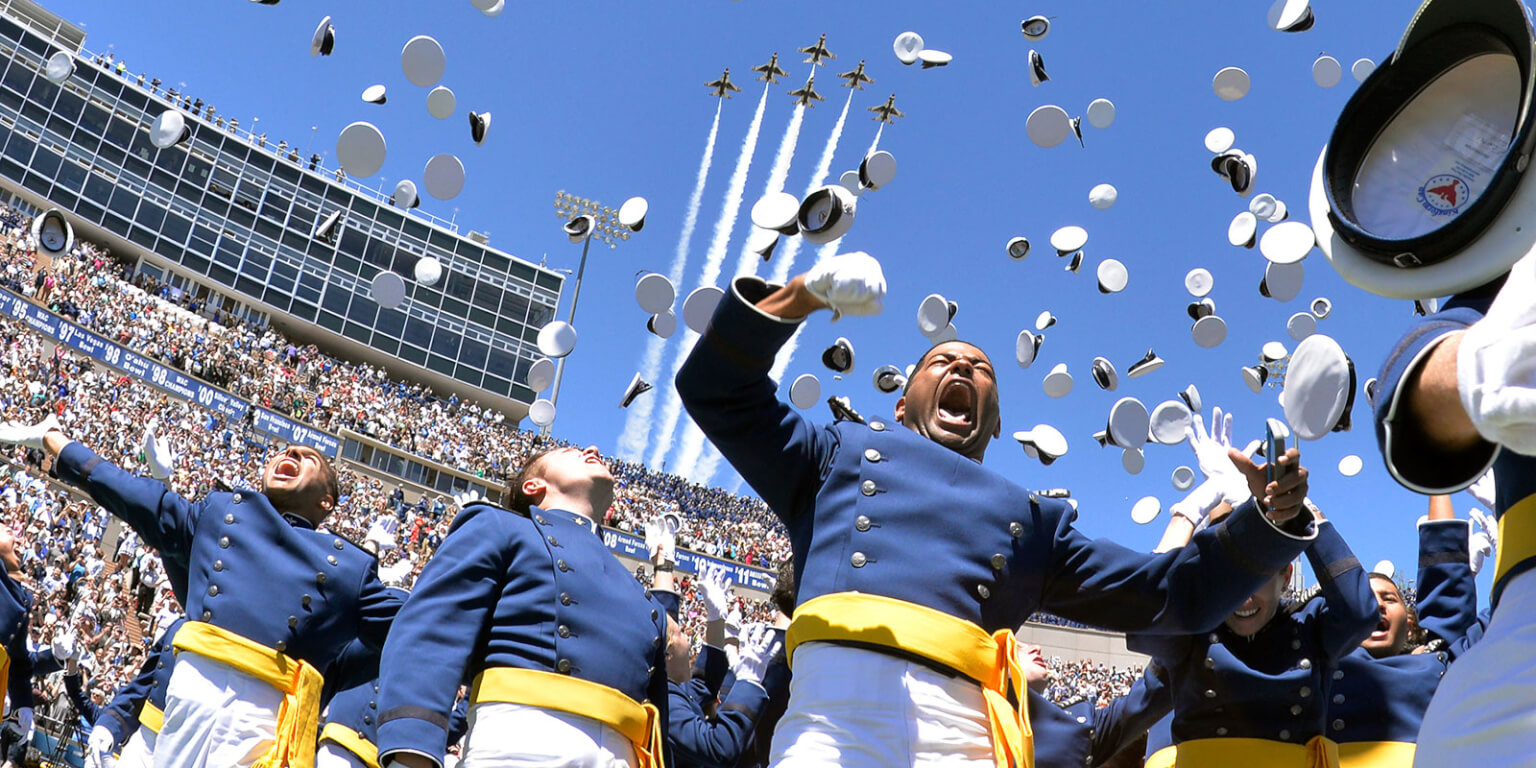In this vibrant and dynamic image, a grand military graduation ceremony or significant event such as the Army-Navy game is in full swing in a packed stadium. The focus is on several young Marines, easily identifiable by their crisp blue jackets adorned with yellow sashes, white pants, and white gloves. The celebratory atmosphere is punctuated by countless white Marine hats being joyously thrown into the clear, cloudless blue sky. Above the scene, a thrilling flyover by six fighter jets adds to the high-energy ambiance, symbolizing precision and might. The main Marine at the forefront, captured mid-celebration with his arms triumphantly raised and mouth open in a yell of victory or exhilaration, epitomizes the collective excitement of the moment. The stadium, bustling with spectators and fellow soldiers alike, provides a robust backdrop to this emotionally charged and visually striking event.